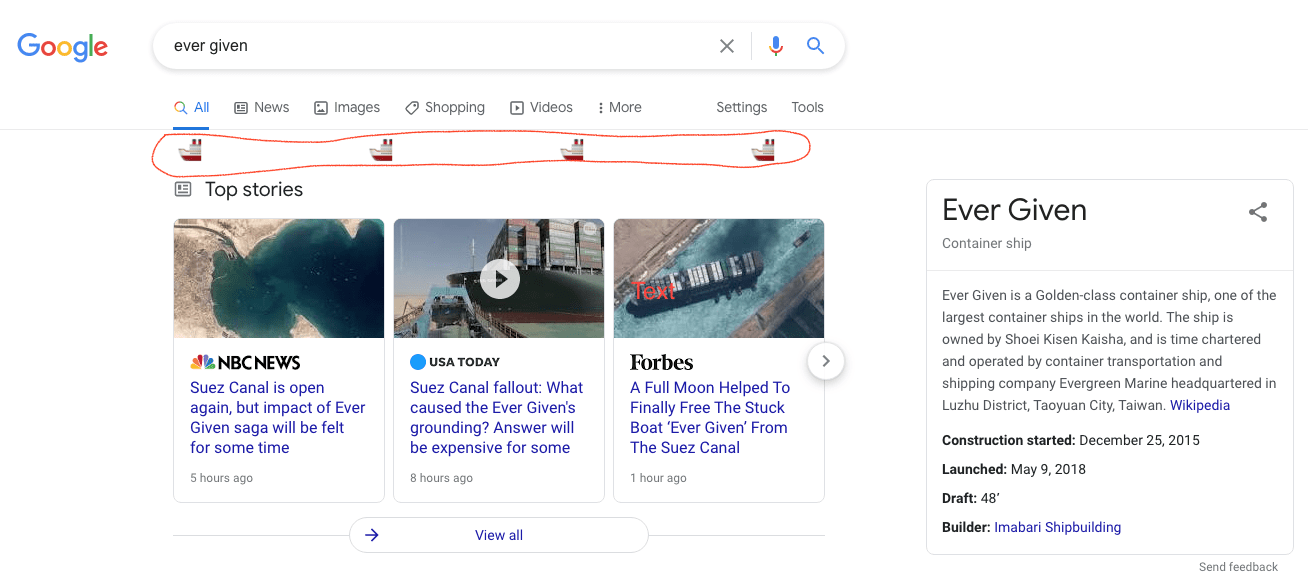This image captures a laptop screen displaying a Google search results page for "Ever Given." In the top left corner, the Google logo is prominently featured in its iconic colors: blue G, red O, yellow O, blue G, green L, and red E, set against a white background. To the right of the logo, there is a search bar filled with the query "Ever Given" in black text. Adjacent to the search bar on the right are three icons: a blue search icon, a blue microphone icon for voice search, and a black X for clearing the search query.

Below the search bar, outside its confines, lies a small magnifying glass icon followed by the word "All" in blue, underlined, indicating it is the selected tab. To the right of "All" are the tabs for "News," "Images," "Shopping," "Videos," and "More" in black. On the far right, the options "Settings" and "Tools" are displayed in black text.

The main content of the screen begins with an image of the front half of a ship, its top painted white and the bottom red, adorned with two red smokestacks visible at the top. The ship is encircled in red ink, drawing attention to it. Beneath this image, a small newspaper icon precedes the text "Top Stories."

The "Top Stories" section features three vertically aligned rectangles, each containing a news article. The first rectangle showcases an image of water spanning from right to about two-thirds of the way left, transitioning into land. Below this image, the NBC News logo sits beside text providing four lines of information, with a timestamp indicating the article was published five hours ago.

The second rectangle displays an image of shipping containers on a dock. Beneath this, the USA Today logo appears above four lines of information, noting the article was uploaded eight hours ago.

The third rectangle hosts an image of water flowing from the left up to the right with concrete structures in the top left and bottom right corners. Forbes is identified below the image, accompanied by four lines of information in blue text, and the article is timestamped one hour ago.

At the bottom center of the screen, a white tab titled "View All" in blue text is present, suggesting the user can access more articles. To the left of this tab, an arrow pointing to the right invites further navigation.

This comprehensive description captures the layout and details of the Google search results page for "Ever Given" as displayed on the laptop screen.